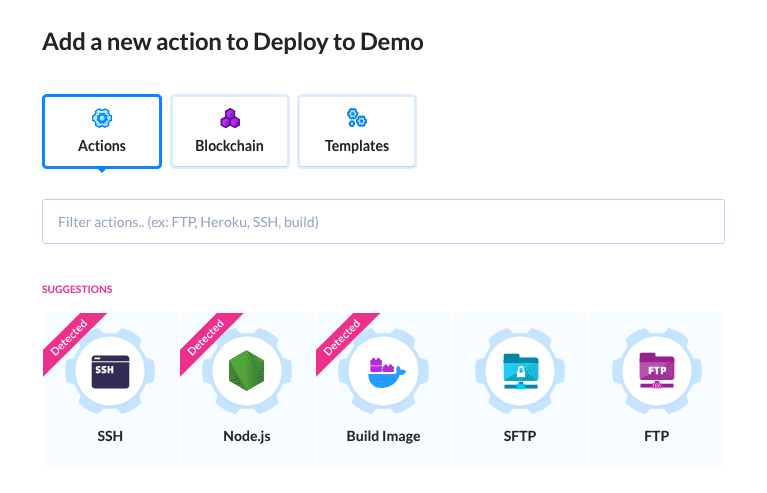The image features a vivid, black title situated in the top left corner that reads, "Add a New Action to Deploy to Demo." Directly below this title, there are three distinct buttons aligned horizontally towards the upper-left quadrant of the page. The leftmost button is labeled "Actions" and is accompanied by an icon resembling a gear. Adjacent to it, the middle button is titled "Blockchain" and features an icon displaying three interlocking shapes colored in purple. The rightmost button, named "Templates," showcases an icon comprising three interlinked gears.

Beneath these buttons lies a search bar with the placeholder text, "Filter Actions." Under this search bar, the page presents five separate action suggestions. Each suggestion is clearly labeled: "SSH," "Node.js," and "Build Image" are marked with the tag "Detected." The last two suggestions, "SFTP" and "FTP," do not have any detection labels. Each of these action names is positioned at the bottom of their respective sections, providing a clear and organized overview for the user.